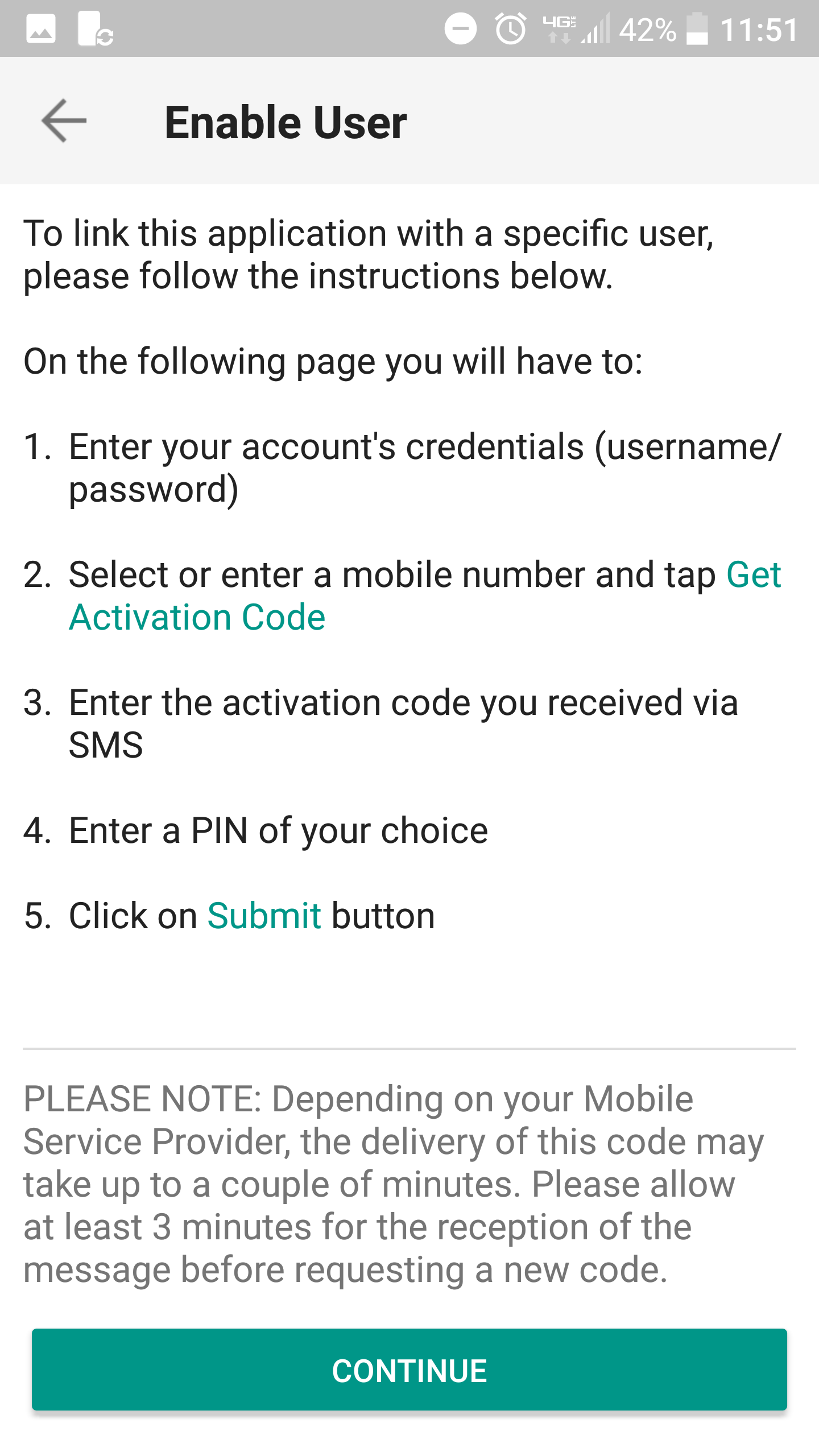Title: User Activation Page on Mobile App

Caption: The image displays a mobile app screen dedicated to enabling a user account. The aspect ratio of the screen is roughly 2.5 times taller than it is wide. At the very top, a slim, gray status bar stretches horizontally, containing standard smartphone icons for alarm clock, 4G signal, Wi-Fi connection, battery status (at 42%), and the time (11:51). Toward the upper left, there are two icons, presumably shortcuts for apps.

Beneath the status bar is a light gray navigation bar, approximately twice the height of the status bar. This bar includes a black back arrow pointing left and bolded text stating "Enable User." This indicates the user is in the activation section of the app.

The main background of the screen is white, featuring black instructional text. The instructions guide the user on linking the application with their account:

1. Enter your account credentials (username and password).
2. Select or enter your mobile number and tap the "Get Activation Code" button in green.
3. Enter the activation code received via SMS.
4. Create and enter a personal PIN.
5. Click the "Submit" button in green.

At the bottom of the screen, a disclaimer is noted, followed by a prominent green button labeled "Continue" in white text.